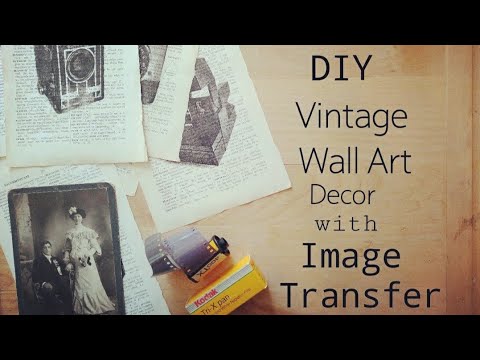The image appears to be a composite art piece likely originating from an advertisement or an instructional video about creating DIY vintage wall art decor with image transfer. The left two-thirds of the image display several printed pages that resemble dictionary entries, each adorned with superimposed pictures of old-style cameras, including vintage Kodak models and a modern Polaroid. At the bottom left, there is a black-and-white antique photo of a man seated in a tuxedo and a woman in a fancy white dress adorned with a flowered hat, standing beside him. The center of the image features a Kodak Tri-X Pan film roll with the film partially pulled out of the canister, and directly below it sits a yellow and white Kodak box. The right-hand side of the image, set against a light wooden background, contains the text "DIY Vintage Wall Art Decor with Image Transfer" in black lettering. The entire composition is laid out on what appears to be a cardboard or a wooden table.